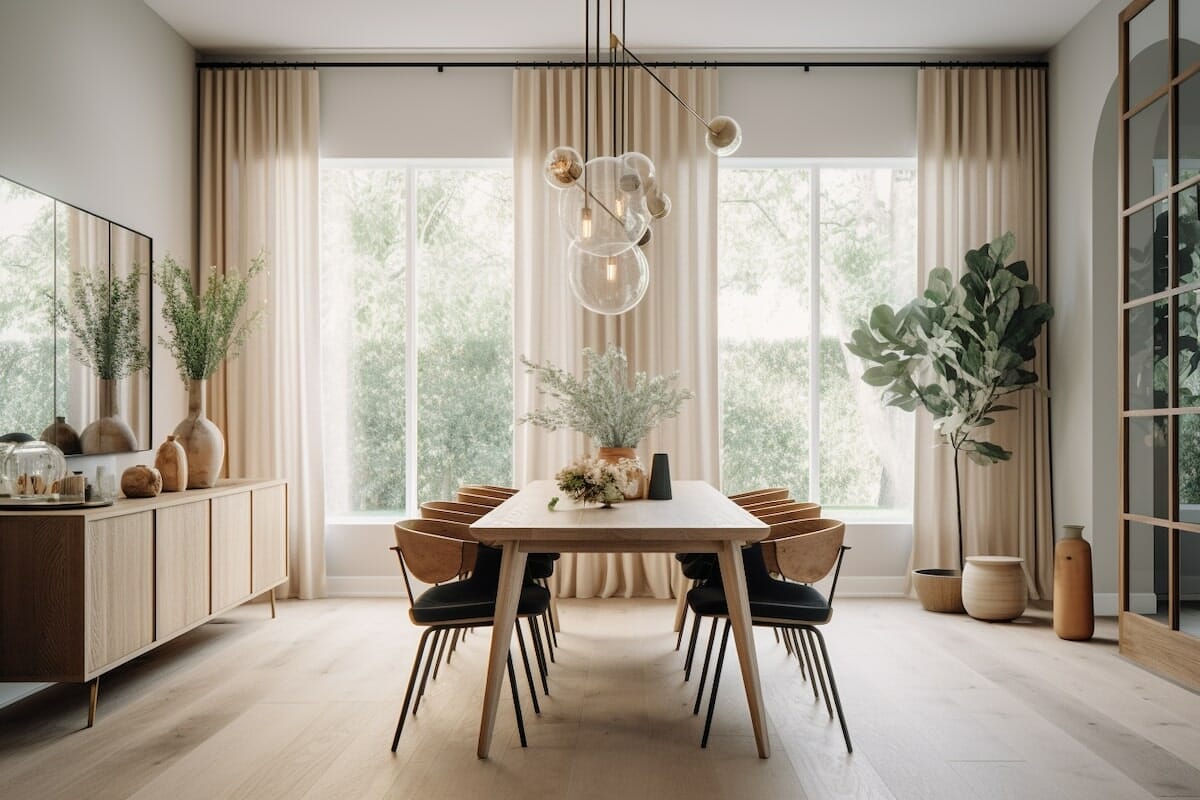The image is a 3D color rendering illustration of a clean, modern dining room. The room features a central light-colored wooden dining table, likely wooden and measured approximately 70 feet in length. This table is surrounded by eight chairs—four on each side—with modern design elements: brown curved wooden backs, black cushioned seats, and black iron legs. On the table, there's a red clay vase filled with white dried flowers, along with a few other accessories.

The room boasts a light wood laminate floor, and walls painted in light gray tones. Prominent in the room are two tall picture windows, one on each side, draped with floor-to-ceiling cream-colored curtains on a black rod spanning the room's width. The windows feature vertical panes and bring a lot of natural light into the space.

A variety of lighting fixtures hang from the ceiling, including modern pendant lights with transparent glass globes and round golden bulbs. An artificial tree and a planter sit in the right corner, accompanied by two vases.

On the left side of the room, there's a low, light-colored cabinet with short legs and sliding doors, topped with three ceramic vases—the largest of which holds greenery. Above this cabinet, a mirror is affixed to the wall.

In additional architectural detail, there is a trellis wall with an arch opening on the right side, ostensibly leading to another room. Overall, the room combines elements of white, tan, gray, black, brown, and green, contributing to a cohesive and stylish atmosphere.